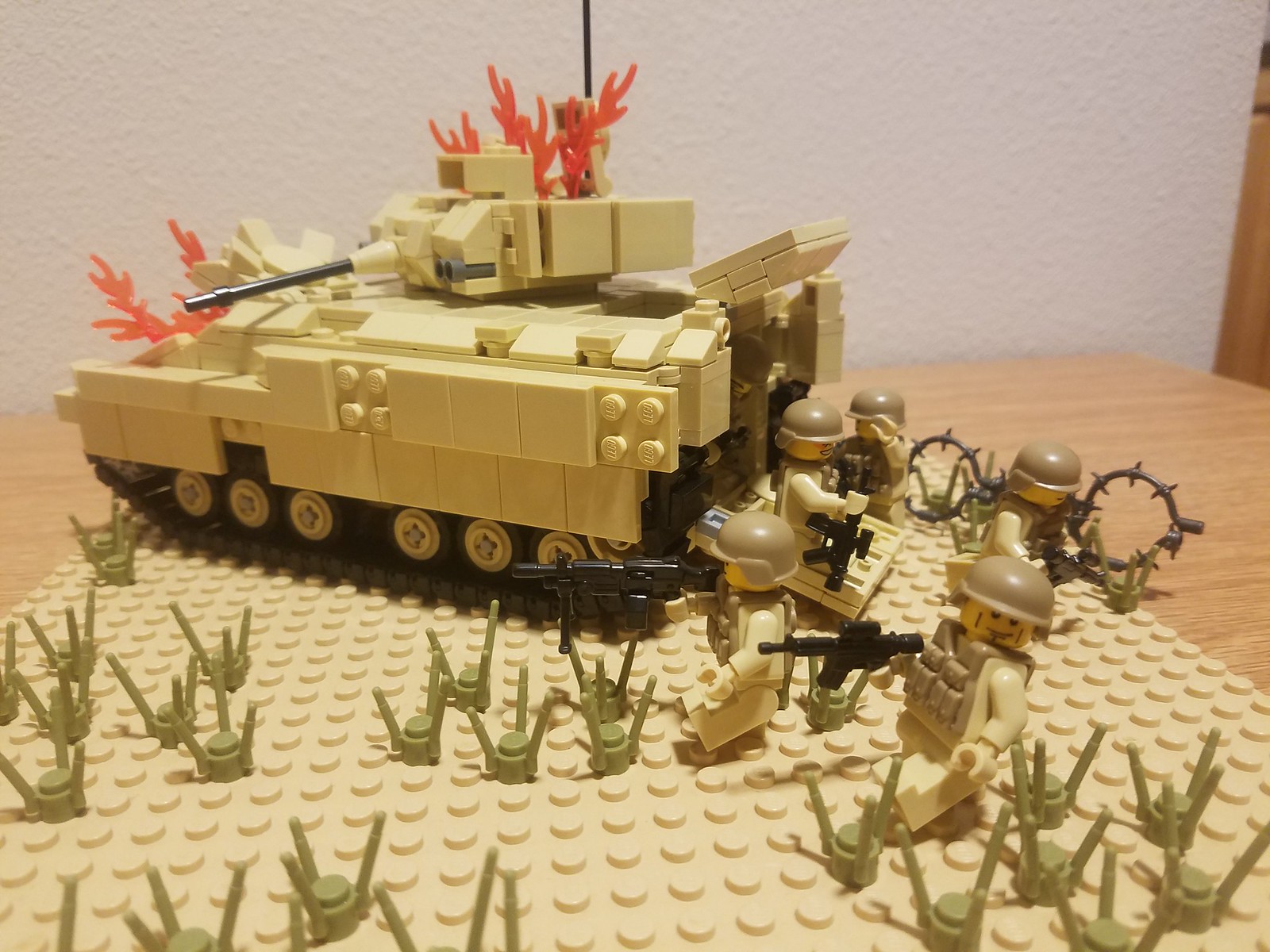This detailed photograph captures a meticulously constructed Lego military scene set atop a light brown wooden table, with a white wall serving as the backdrop. Central to the image is a tan-colored Bradley fighting vehicle built from Legos, which is depicted in a state of distress with vivid red and orange Lego flames emerging from its top. The Bradley, made up of many standard Lego pieces, has its back ramp open and turret slightly turned to the side, suggesting action and urgency.

Surrounding the Bradley is a detailed tan Lego platform, sporadically adorned with small green three-pronged Lego pieces that resemble grass. Emerging from the back ramp and scattered around the platform are six miniature Lego soldiers, designed with intricate details. These soldiers are outfitted in military helmets, bulletproof vests, and are equipped with black rifles and machine guns. They are depicted in motion, seemingly evacuating the vehicle due to the fire.

The combination of tan, olive drab green, and black colors on the soldiers adds to the realism of the military scene. The image captures the precision and creativity involved in assembling such an intricate Lego set, emphasizing the chaotic yet organized environment of a military scene under duress. The overall composition effectively conveys a dramatic narrative of soldiers evacuating a damaged vehicle amidst a fiery chaos.